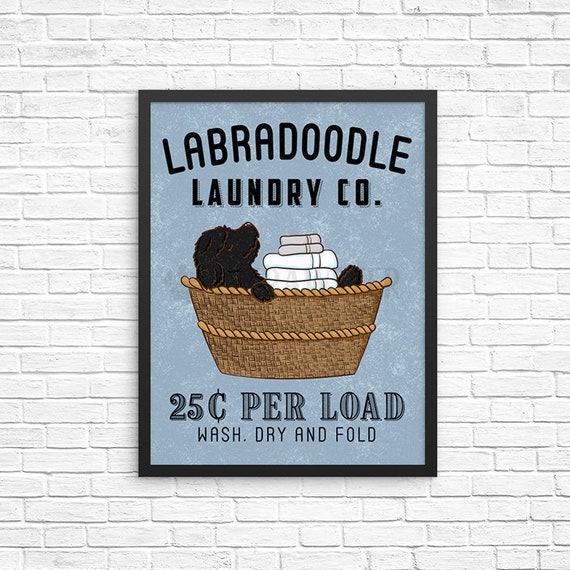The image is a photograph of a charming and whimsical advertisement for the Labradoodle Laundry Company. The sign, framed in black, features a serene labradoodle puppy reclining in a woven brown basket with a neat stack of clean towels and washcloths resting on its chest, adding to the relaxing and cozy atmosphere. The background of the sign is a light blue color, contributing to its clean and inviting aesthetic. The wording on the sign states "Labradoodle Laundry Co.," followed by "25 cents per load, wash, dry, and fold," hinting at laundry services provided at an impressively low rate. The sign is mounted on a white-painted brick wall, which enhances the overall sense of cleanliness and charm. This pleasant and decorative piece could be found in a laundromat or someone's laundry room, adding a cute, fun vibe to the environment.